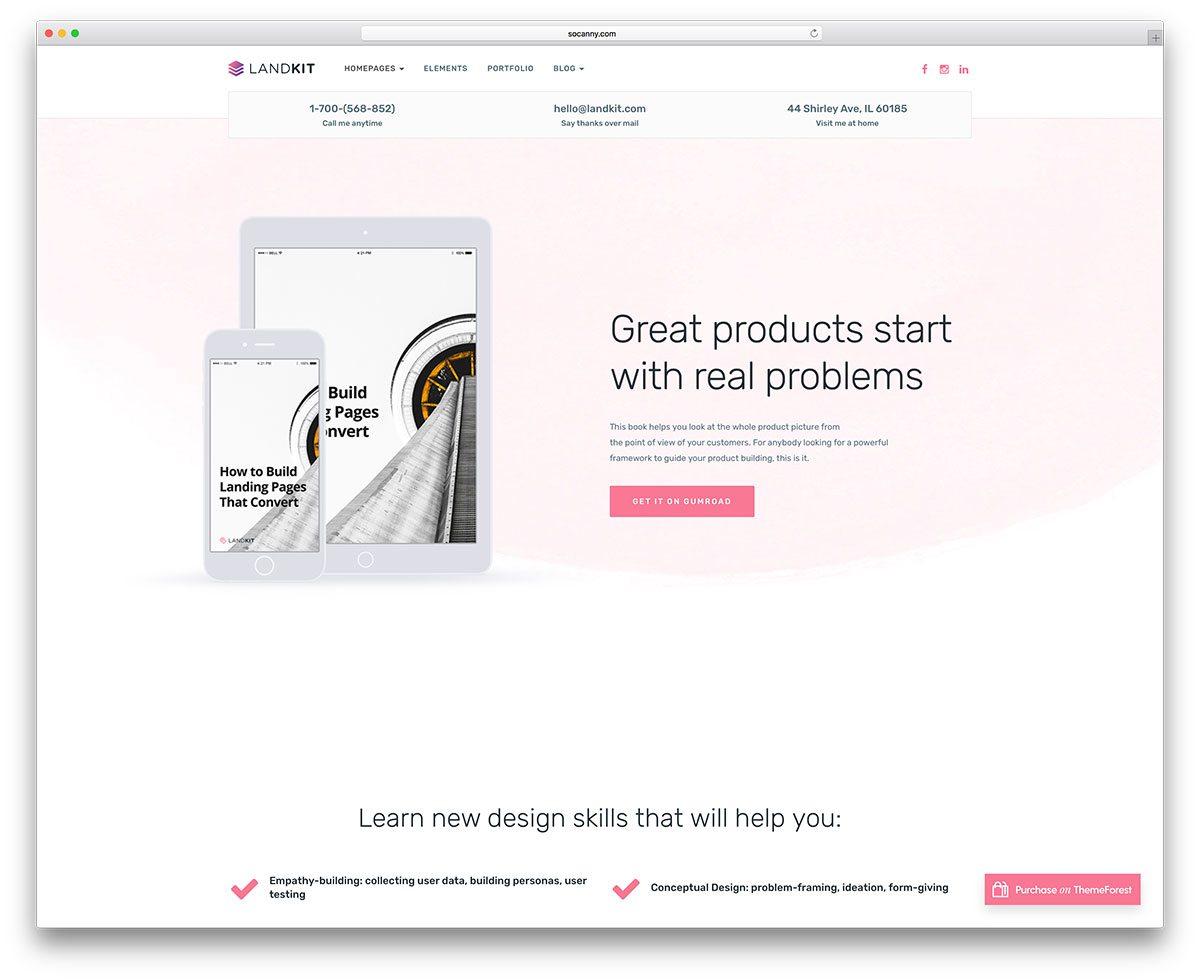The image depicts a webpage viewed on what appears to be an Apple device, likely identifiable by the characteristic interface elements such as the red, yellow, and green dots typically seen on the left side of an open window. The website featured is soulcandy.com, with the branding for "LandKit" prominently displayed. The navigation menu includes options for Home Pages, Elements, Portfolio, and Blog. 

To the right side of the page, the social media icons for Facebook, Instagram, and LinkedIn are displayed, followed by contact information in pink letters: "Call anytime: 1-700-568-852" and "Email: hello@landkit.com". There's also a playful invitation with phrases like "Say thanks over mail" and "Visit me at home" alongside the address "44 Shirley Avenue, Illinois, 60185".

A highlighted message states, "Great products start with real problems. This book helps you look at the whole product picture from the point of view of your customers." It promotes a book beneficial for those seeking a powerful framework to guide their product building efforts, available on Gumroad. The book aims to teach new design skills including empathy building, collecting user data, building personas, user testing, conceptual design, problem framing, ideation, and form giving—each item followed by a check mark.

Finally, there is a prompt to "Purchase on ThemeForest," indicating that the overall objective is to facilitate the purchase of the product or service being featured.